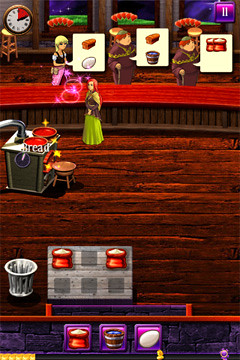In the video game scene, a woman with red hair is dressed in a green dress, engaging in conversation with an individual who has yellow hair. The person with yellow hair requests a loaf of bread and an egg. Nearby, there is a portly man in a brown robe with red hair, who desires a loaf of bread and a bucket of water. Beside him is another identical portly man in a brown robe with red hair, who is asking for two bags of rice.

In the scene, a small silver oven is visible, containing a fire. Atop the oven are two pots filled with a red substance. Below the oven sit two bags of rice. Adjacent to the oven, there is a trash can. Below this setup, another bag of rice, a bucket of water, and an egg are positioned. In the top left-hand corner of the screen, a clock is displayed with a section highlighted in red, indicating the passage of time.

This detailed description captures the intricate demands of the characters and the various elements present in the game scene.